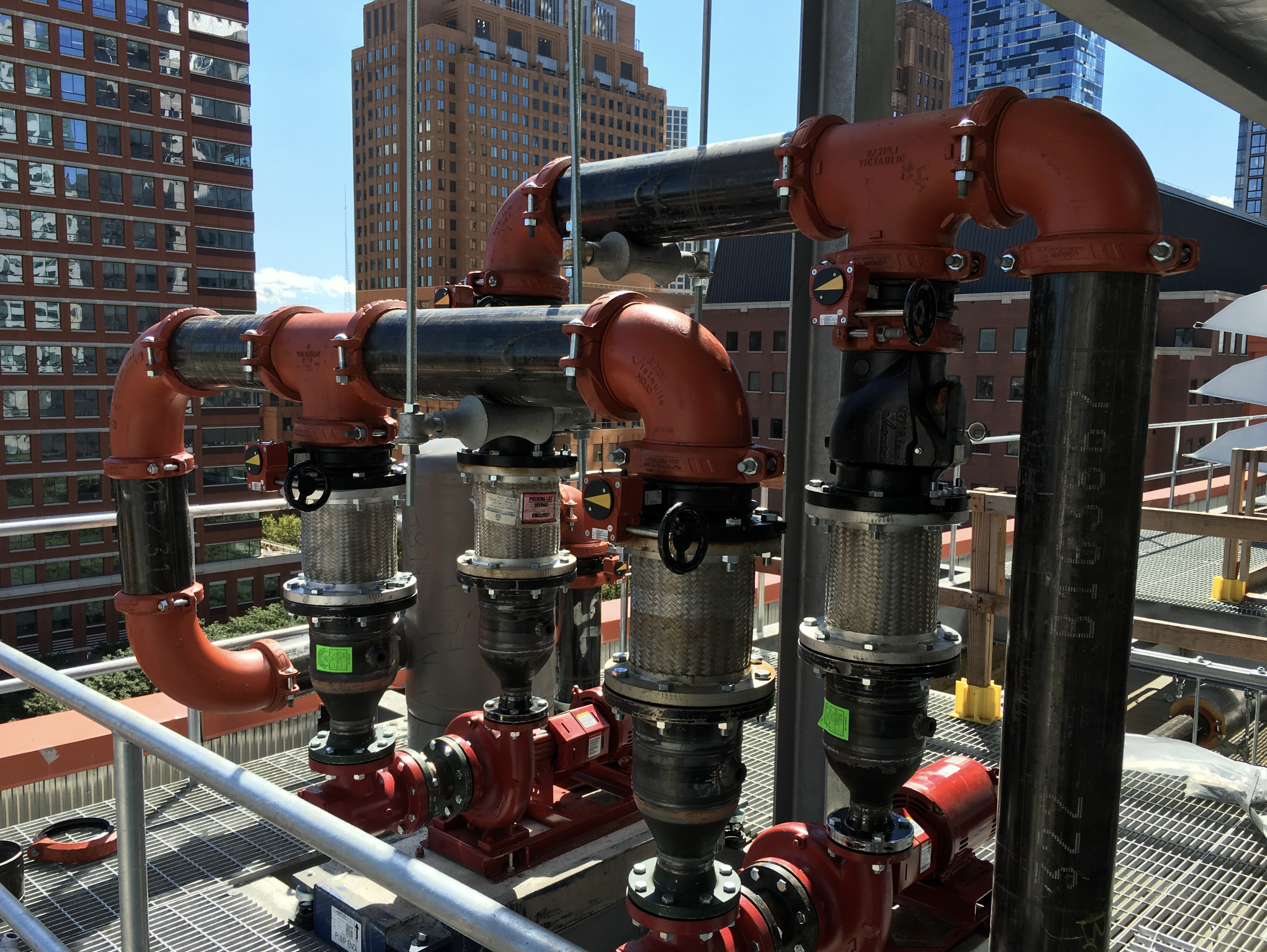This is an angled view of a sophisticated pump system located on the rooftop of a city building. The system features black pipes with red curved accents, connected to a red machine, all mounted on a silver grate platform. Surrounding the platform are round metal fences that provide safety on the roof. The primary pipes, connected in an upside-down U-shape, also include chrome accents and black valves, highlighting their functional design. To the left in the background, towering red skyscrapers with many windows rise high, their glass reflecting the bright blue sky dotted with a few small white clouds. To the right, another metal platform with metal fences is visible, contributing to the urban industrial scene.